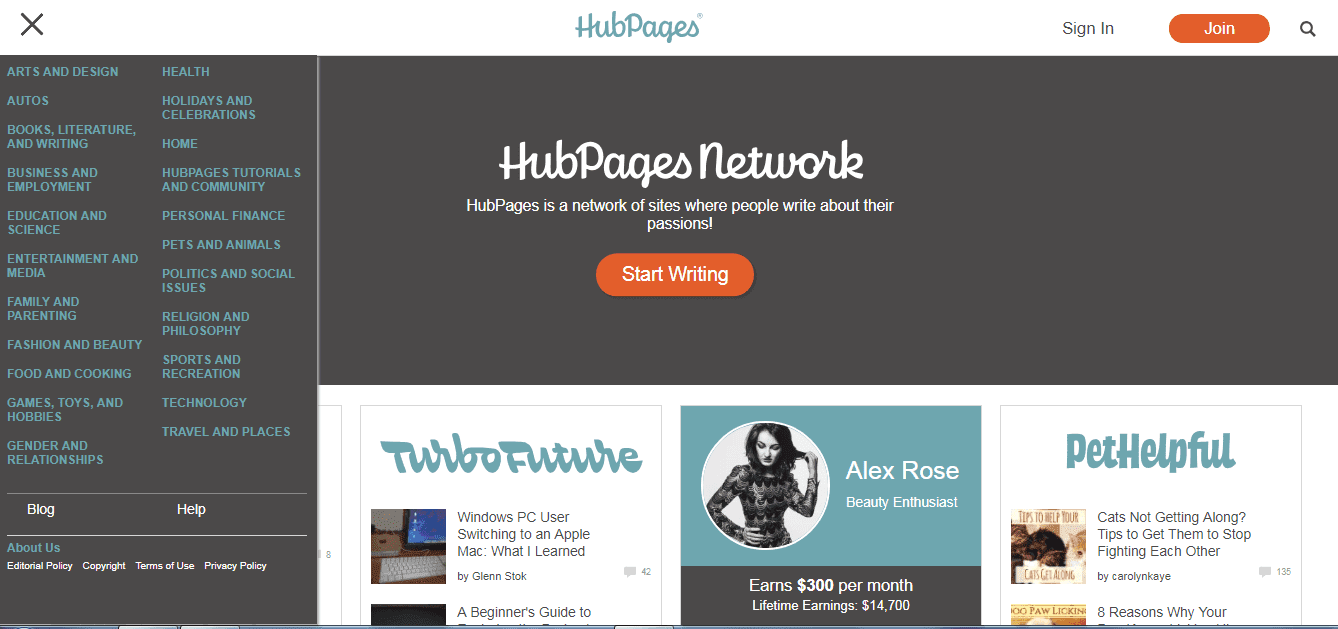This screenshot features a user interface from the HubPages website, set against a gray and white background and formatted in a horizontal layout. In the upper left corner, a white header displays a gray "X" on the left side, and the name "HubPages" is styled in blue cursive text at the center. On the upper right, "Sign In" is written, followed by a prominent orange "Join" action button.

Below this header, white text on a gray background reads "HubPages Network," introducing HubPages as a collection of sites where individuals write about their various passions. An orange "Start Writing" action button in white text is prominently displayed below this brief description.

To the left, a dark gray box contains a vertical list of topics, each in blue text: Arts and Design, Autos, Books, Literature and Writing, Business and Employment, Education and Science.

In the lower right corner, there is a circular photo of a woman shown from the waist up. To the right of this image, text identifies her as "Alex Rose, Beauty Enthusiast."